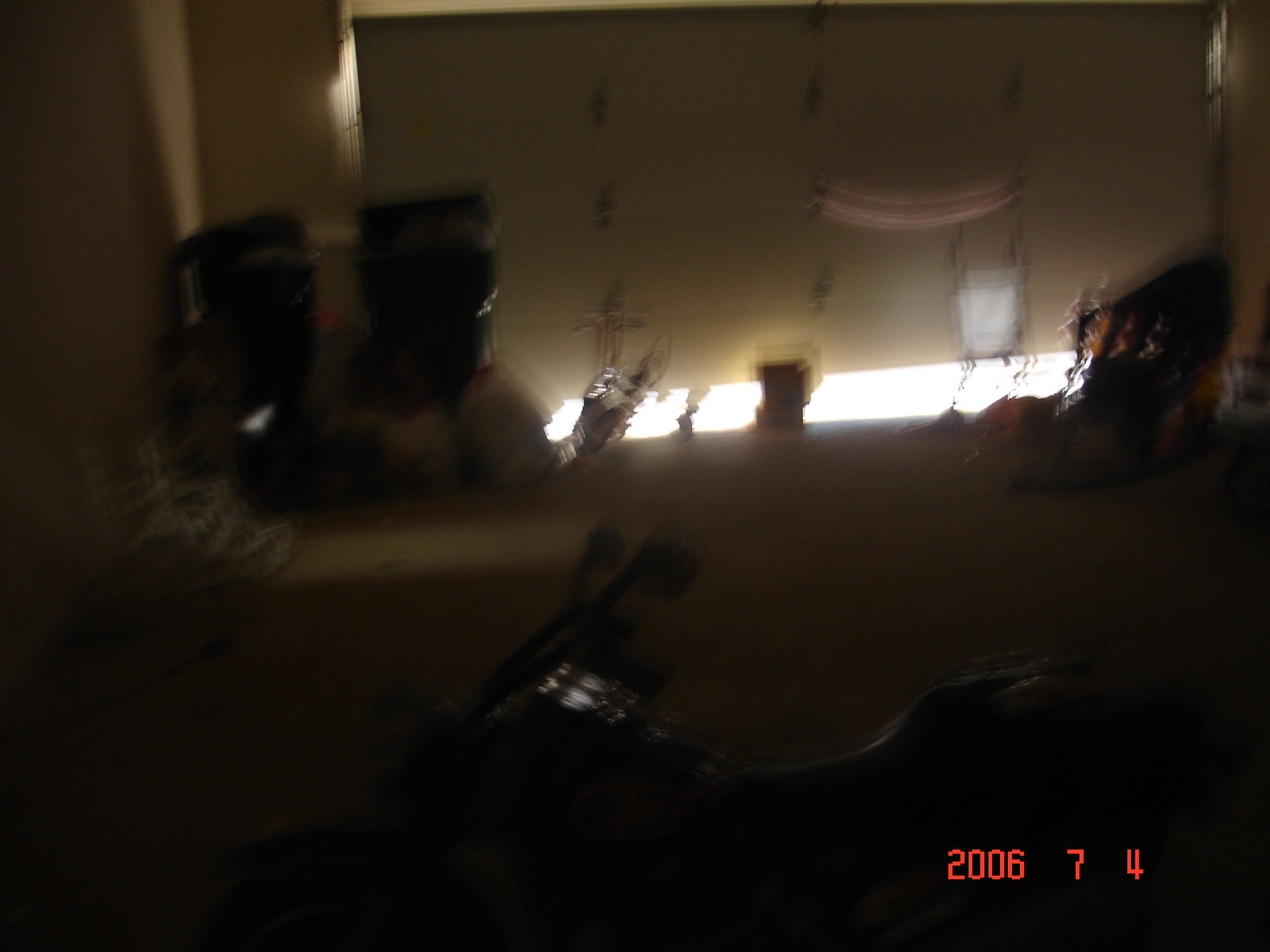The image depicts a dimly lit bedroom with a window partially obscured by a dresser, allowing only slivers of bright light to penetrate the room. Various objects fill the space, contributing to a somewhat cluttered appearance. On the left side, several large black items rest atop bags, with a cross positioned nearby. Toward the right, an odd, elongated black object adds to the room's mysterious ambiance. Closer to the camera, the silhouette of a toy motorcycle can be seen, distinguished by a metal rod on its side. A red date, "2006 7 4," is displayed in the bottom right corner of the image.